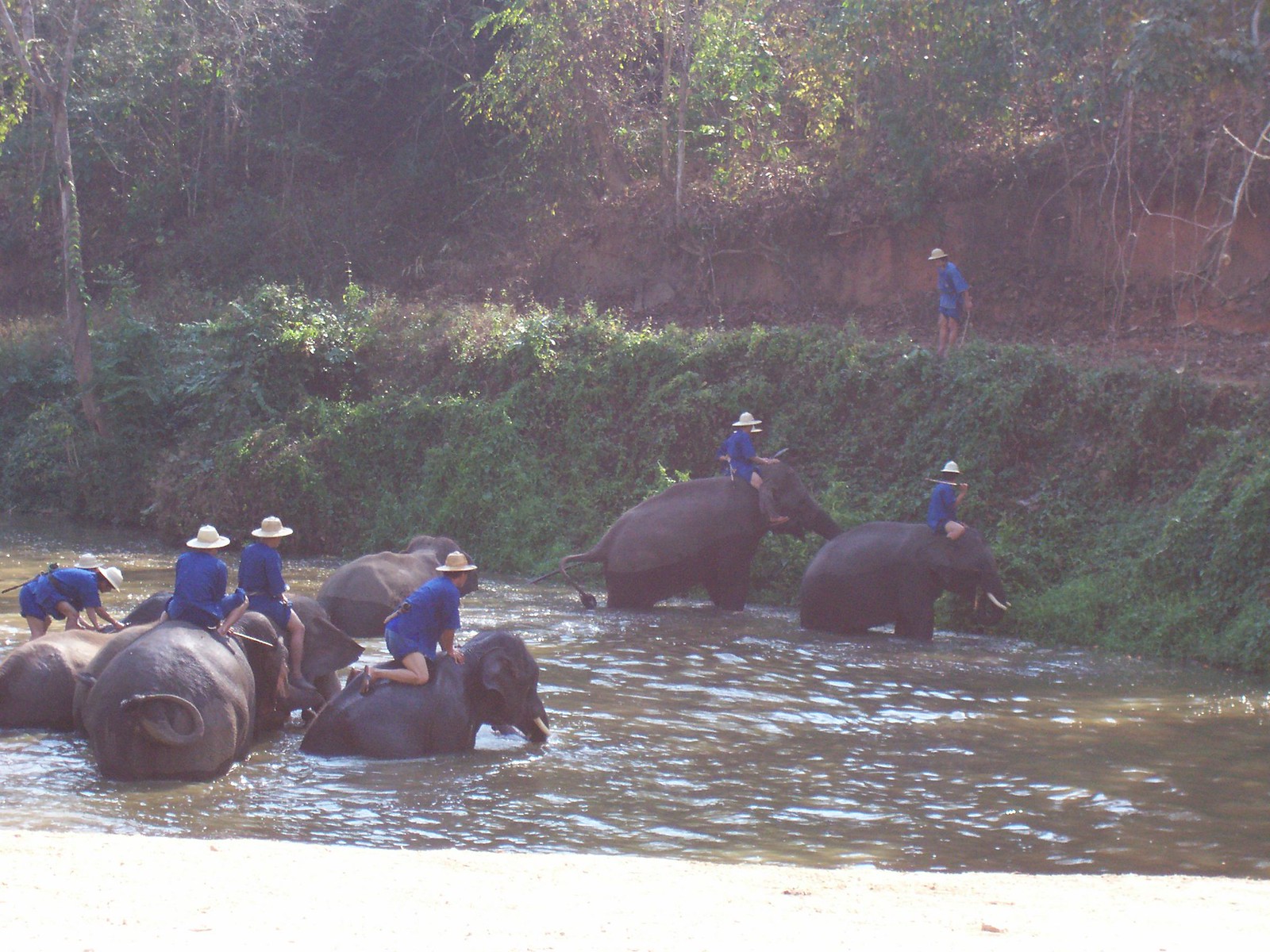This photograph captures a vibrant outdoor scene, showcasing approximately seven elephants wading through a murky brown river with sunlight reflecting off the water's surface. Each elephant is ridden by a person clad in a uniform of blue short-sleeved shirts, blue shorts, and tan safari hats, with one rider equipped with a belt and a rope. The group is moving towards a towering, grassy bluff on the right-hand side, characterized by green, vine-like plants and interspersed with brown dirt. The background reveals additional cliffs adorned with dirt and lush green trees. There's also one person standing atop the bluff, wearing the same attire, observing the scene below.